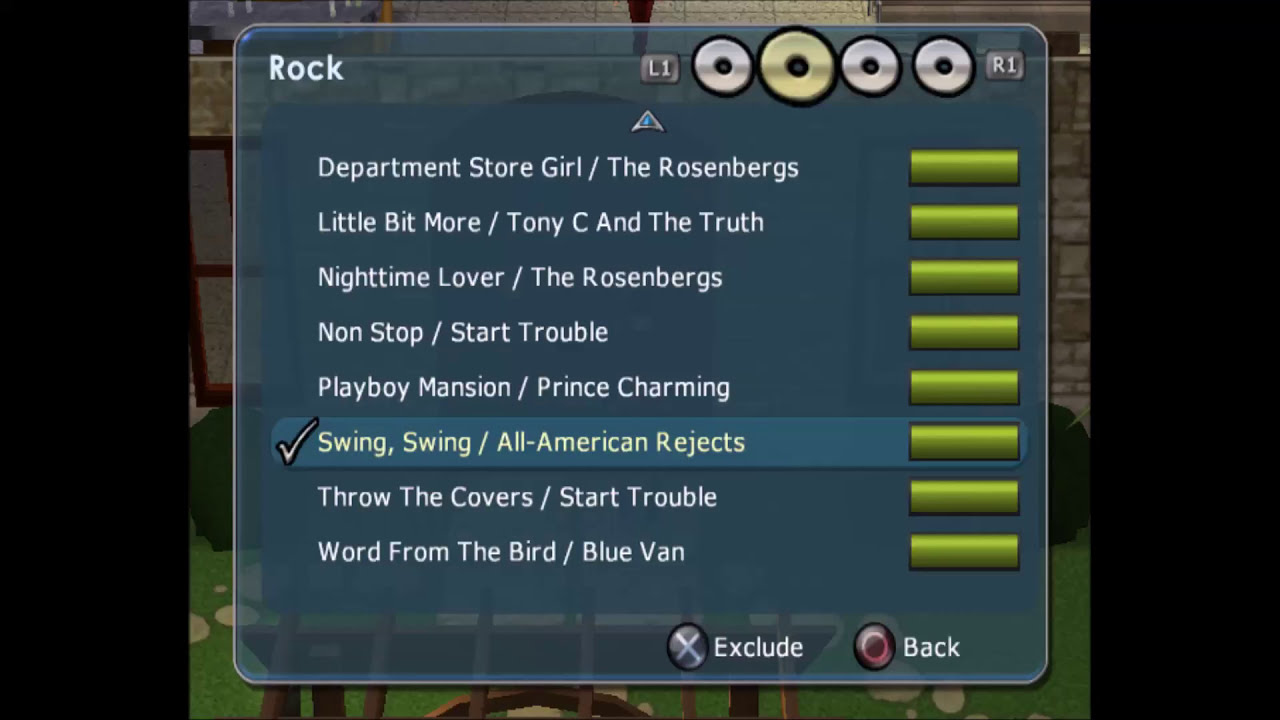The image is a screenshot from a video game interface that closely resembles a 90s-style karaoke screen. The background showcases an illustration that seems to be either a room or the exterior of a building, but it's largely indiscernible. Dominating the screen is a playlist of rock songs in muted monochromatic shades of blue, green, gold, silver, white, red, and black. The top left corner features the word "Rock," accompanied by circular icons resembling control knobs and buttons labeled L1 and R1. 

Below these elements is a text list of songs, starting with "Department Store Girl" by The Rosenbergs, followed by "Little Bit More" by Tony C and the Truth, "Nighttime Lover" by The Rosenbergs, "Non-Stop" by Stark Trouble, "Playboy Mansion Prince Charming," "Swing Swing" by All American Rejects (which is highlighted with a checkmark), "Throw the Covers" by Stark Trouble, and "Word from the Bird" by Blue Van. Each song entry is paired with an oblong green button for selection.

At the bottom of the screen, there are icons for navigation: an X next to "Exclude" and a red circle next to "Back." The overall feel of the interface invokes the ambiance of being in a karaoke bar after midnight, selecting songs to sing, bathed in the nostalgic hues of muted blues and greens.